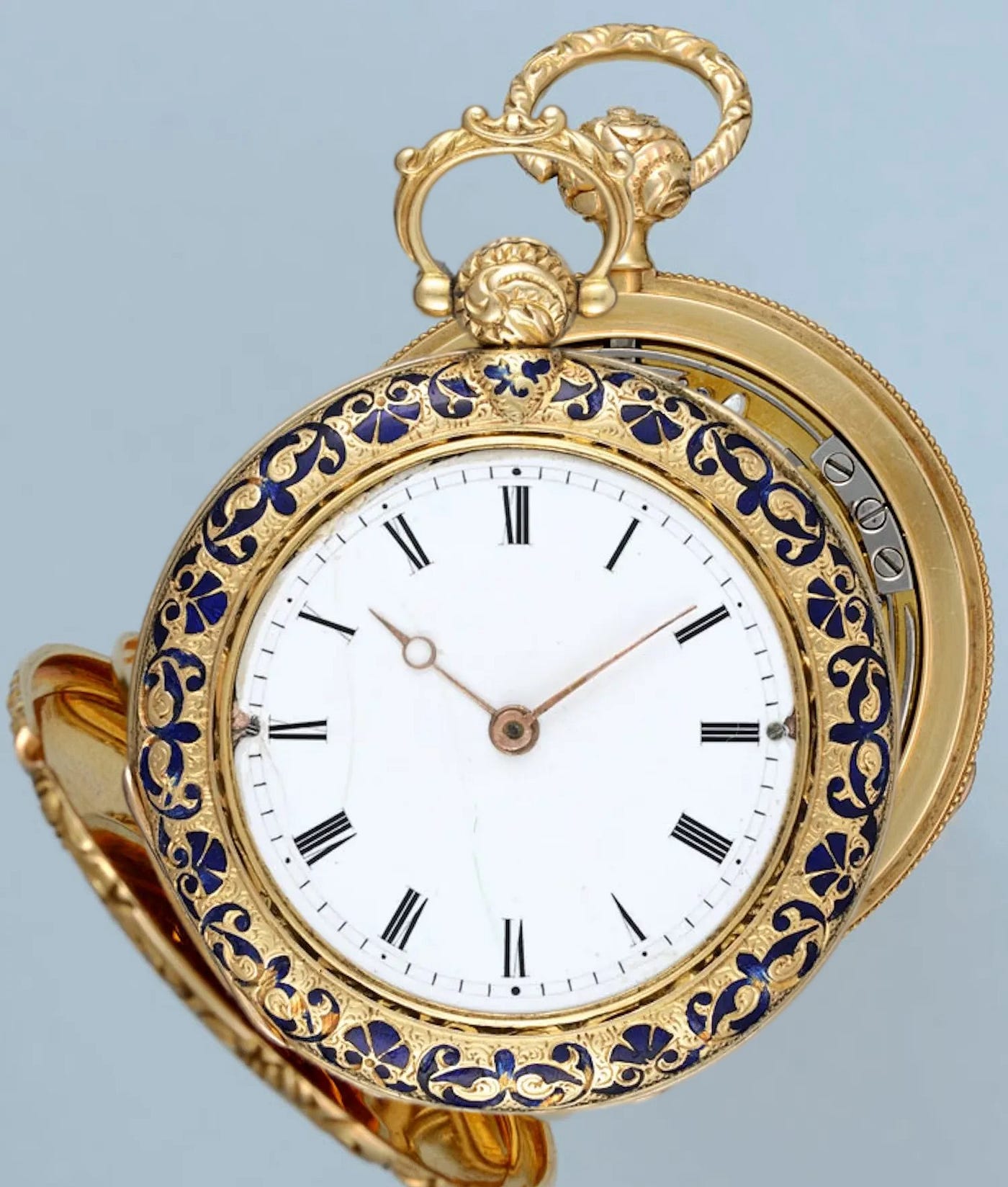This vertical rectangular image captures a close-up of a vintage pocket watch set against a grayish blue background. The pocket watch itself is an exquisite piece, predominantly gold with intricate detailing. The face of the watch is white, adorned with black numeral numbers, and shows the time as 10:10. The hour hand is straight while the minute hand features a loop at its end, adding to the intricacy. Surrounding the watch face is a dual-colored border in gold and dark blue, which hints at artistic craftsmanship. Notably, there seems to be an outer cover in gold, partially visible at the lower left corner, which encases the watch, and another dark-backed piece adds to the complexity. Topping the watch is a fancy gold loop connected to a gold ball, adding both functionality and aesthetic appeal. The image effectively highlights the shine and detailed artwork, showcasing three distinct parts: the main time-telling piece, an additional part for clicking it open, and the mechanism that holds it together. This portrayal of the pocket watch emphasizes its historical charm and intricate design.